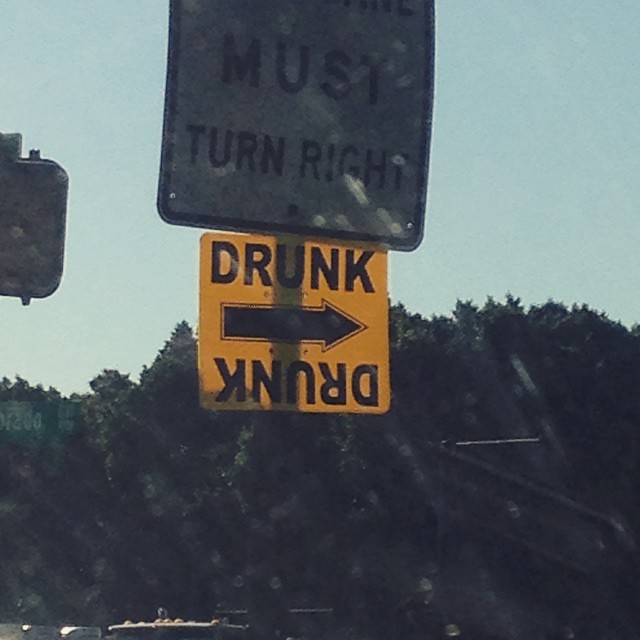In the image, there is a yellow sign prominently featuring an arrow pointing to the right with the word "DRUNK" spelled out clearly on the top. Below "DRUNK," there is an intriguing set of characters spelling "KNERD" with the letters appearing as if they are partly upside down and reversed: a backward, upside-down "K," an upside-down "U," a backward "R," and a backward, upside-down "D." 

Above this yellow sign, there's a slightly rectangular white sign with the command "MUST TURN RIGHT" spelled out letter by letter. The sky is dotted with white, floaty particles, adding a whimsical element to the scene. In the background, you can see lush green trees, providing a natural backdrop. In the top left corner of the image, there's a black box with two protrusions on each side, adding an element of mystery to the composition.